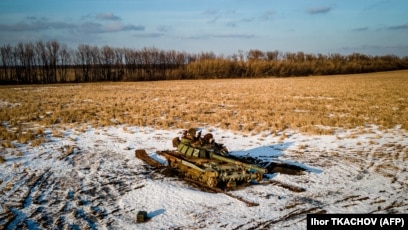The photograph is a blurry image of a flat landscape, where the layout is in landscape orientation, meaning the sides are shorter than the top and bottom. The top third of the image features a light blue sky with some cloud coverage. Below that, there is about 10% of the image showing a horizon lined with thin, tall trees and orangey-green bushes, appearing dead as if in winter. The midsection depicts a band of brown dead grass or weeds. The foreground is dominated by a clear area covered with what looks like white sand or snow. On this white surface sits a military vehicle resembling a small tank, characterized by a long, protruding cannon and vague shapes suggesting one or two occupants, though the blur makes it hard to discern exact details. A light brown, wooden object that might be a sled is also mentioned. In the bottom left corner, a black banner with white text reads "IHOR TKACHOV (AFP)".